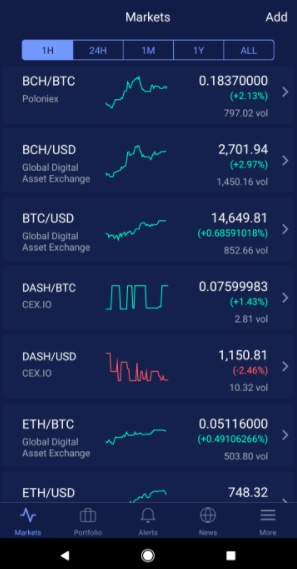This screenshot depicts a mobile app interface related to stock trading or cryptocurrency markets, with a predominantly navy blue background. At the very top center of the screen, "Markets" is displayed in white font, while the word "Add" appears at the top-right corner. Below this, there is a blue rectangular bar featuring time intervals labeled as "1 hour," "24 hours," "1 month," "1 year," and "All," with the "1 hour" option currently selected.

The main content area displays digital currency pairs, specifically:

1. BCH/BTC: 
   - Conversion rate: 0.1837000 (in white font)
   - Percentage change: (2.13%) (indicated in parentheses with an asterisk)
   - Volume: 797.02 VOI

2. BCH/USD (Global Digital Asset Exchange):
   - Conversion rate: 2701.94
   - Percentage change: +2.97% (in parentheses)
   - Volume: 1450.16 VOI